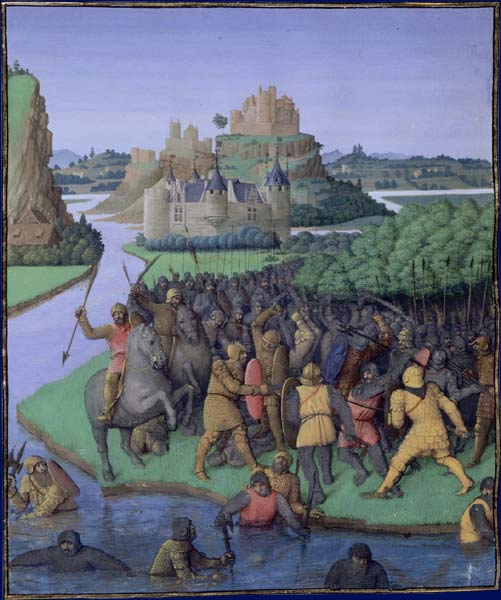The vibrant and detailed image depicts a vivid medieval battle scene. Nestled in the background is a grand castle, with its gray stone structure and black rooftops, situated atop a hill and surrounded by a winding moat or river. The foreground is a bustling battlefield with knights and soldiers clad in protective armor, distinctly dressed in grays and reds, some atop horses brandishing spears and swords, while others engage in combat on foot using shields, pitchforks, and spears. The green field where the battle ensues is dotted with hedges, while the surrounding landscape features lush greenery, hills, and various medieval homes. The sky is painted a deep indigo blue, contrasting with the rich greens of the trees and grass, all contributing to the vivid color palette that includes shades of red, brown, and beige. Soldiers are seen fighting in the water around the castle, indicating a fierce offensive. This meticulously detailed scene evokes a clear and dynamic portrayal of a medieval era battle, filled with action, color, and historical ambiance.